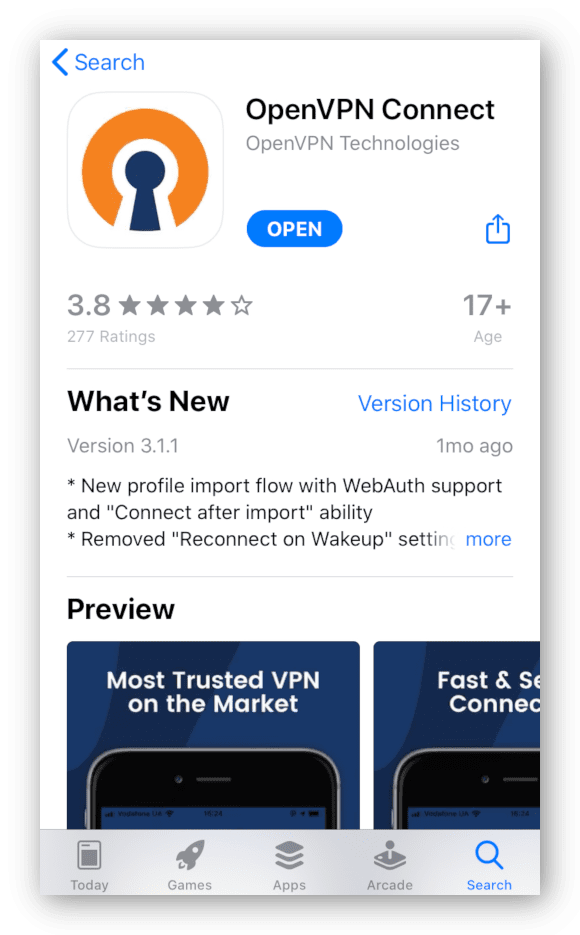The image depicts a clean, white interface reminiscent of an app store or a software download page. Dominating the upper part of the page, a large, centered rectangle showcases details for an application. 

In the top left corner of this rectangle, the word "Search" appears in blue, coupled with a small blue arrow pointing to the left, suggesting a navigation or back button. Centrally positioned within the rectangle is the title "OpenVPN Connect" in bold black text, followed by "OpenVPN Technologies" in smaller black font beneath it.

An illustrative element in the form of a thick, three-quarters orange circle with a white-outlined black lock icon in its center sits prominently within a square outline, adding a visual focus to the description. Further enhancing the interface, a small blue banner displaying the word "Open" in white is situated below the symbol.

To the right, an outlined blue box with an upward-pointing blue arrow contains the version rating "3.8" in gray, accompanied by stars indicating a rating score. Adjacent to this section, "17+" followed by the word "age" labels the application’s age-appropriateness.

Just below, a fine gray divider separates the details. The heading "What's New" appears in black on the left, with "Version History" in blue to the right. Under “What's New,” the text lists updates for version 3.1.1, released one month ago. The updates include a new profile import flow with WebAuth support, a connect after import ability, and the removal of the "reconnect on wake up" setting, indicated with asterisks and quotes. A "More" link in blue offers additional information.

Another fine gray line divides the content below, leading to the "Preview" section in black text to the left. Two blue boxes offer insights into the application features: the first displays the text "Most Trusted VPN on the Market" in white overlaid on an incomplete image of a smartphone. The second features the phrase "Fast and Secure Connect," though it’s truncated by the border of the app’s display.

At the bottom of the page, a gray navigation bar indicates various categories: "Today" with a small square icon, "Games" represented by a rocket, "Apps" with three stacked squares, "Arcade" illustrated with an additional symbol, and finally "Search" in blue alongside a blue search icon. This setup provides a comprehensive yet user-friendly overview of the application and its latest updates.